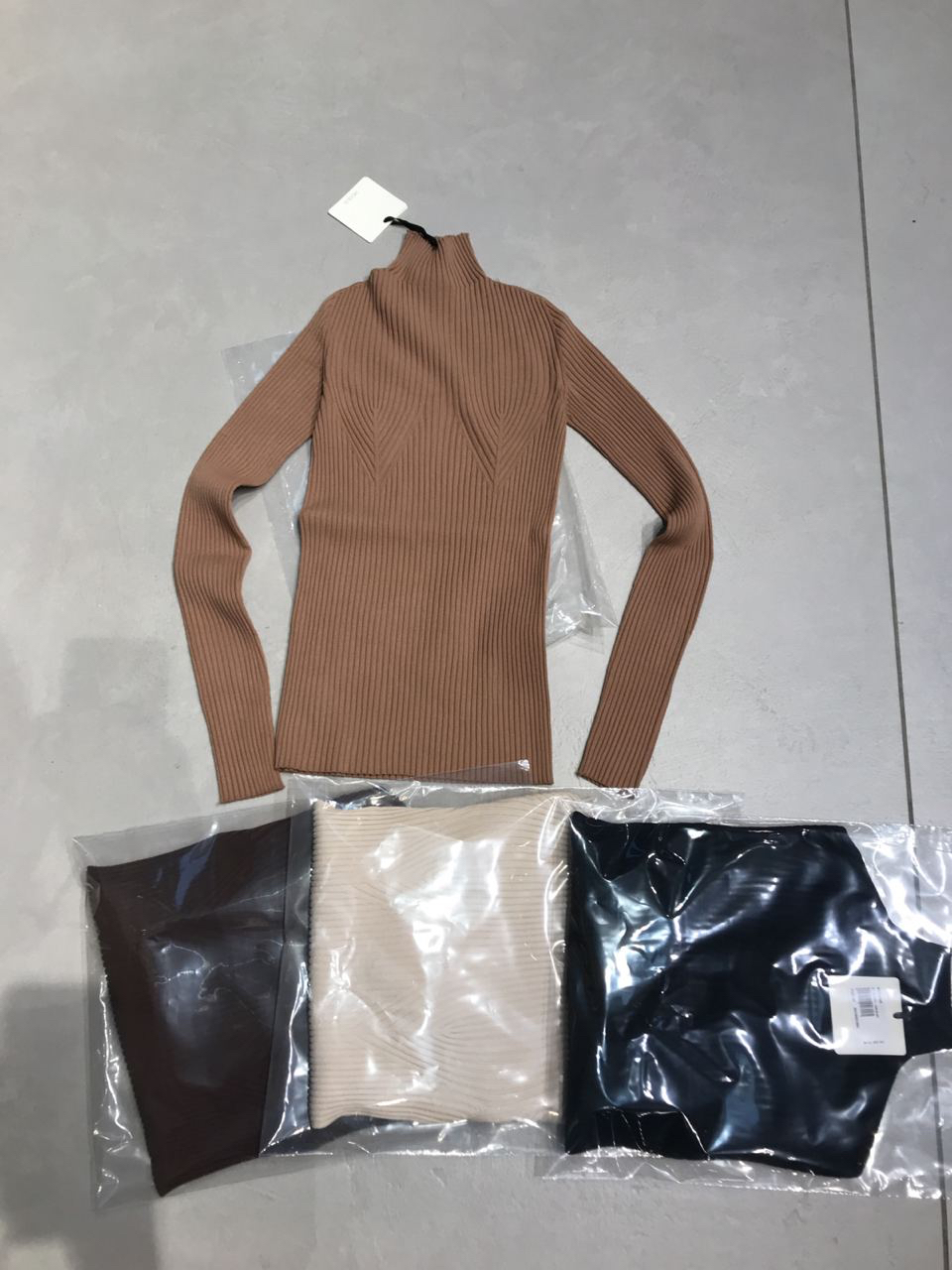The image displays a medium brown, ribbed, long-sleeved sweater with a mock neck, featuring a white tag hanging from the neckline. This sweater lies on a light gray, patterned surface, which could be a table, counter, or possibly the floor, discernible by a large seam or grout line to the right. Beneath the sweater, there are three tightly wrapped and folded garments inside clear plastic bags. The garments are in black, beige, and dark brown/black colors, each similarly packaged with visible tags. The outline of the plastic wrapping underneath the main brown sweater is also visible in the image. The entire setup is photographed in a rectangular format in an indoor setting.